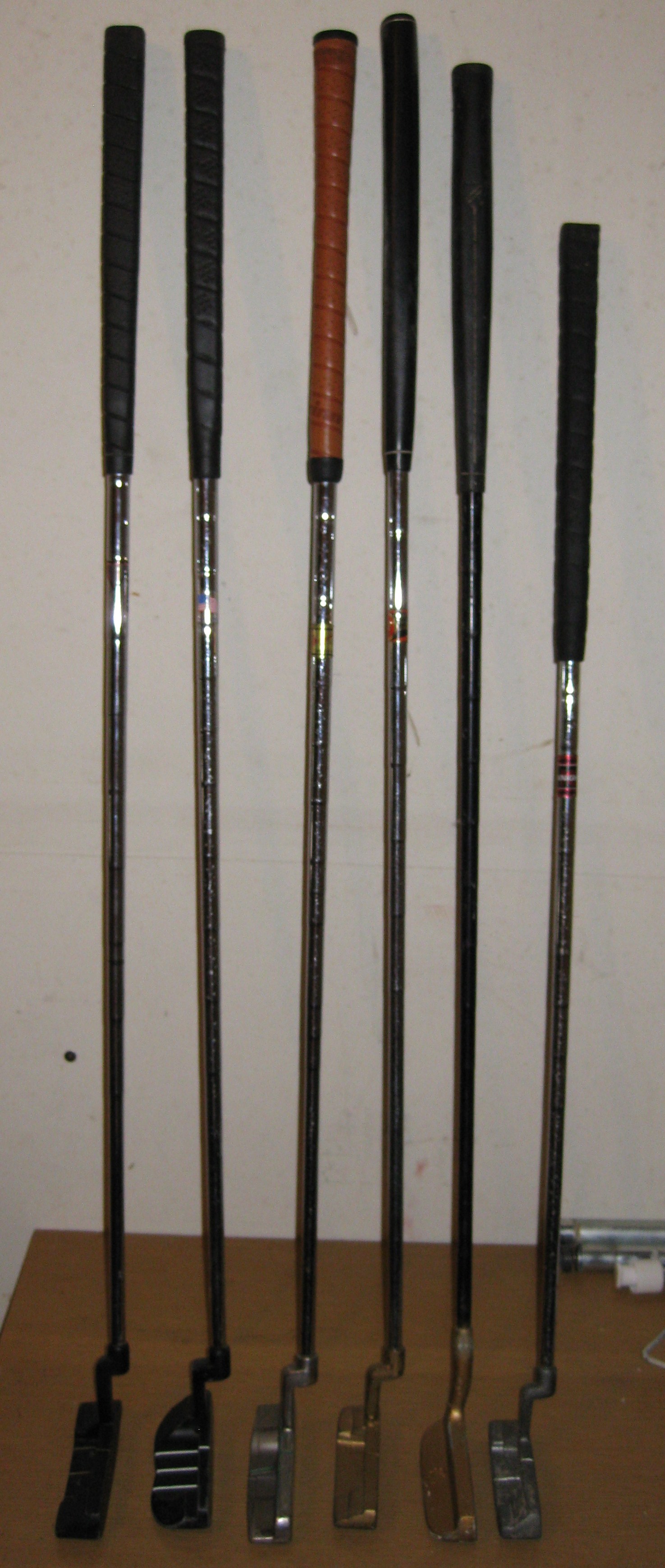This close-up image captures a one-foot-by-one-foot section of a hardwood floor in the corner of a room, showcasing six golf putters leaning against a plain white wall. The putter heads rest on the floor while the handles are propped against the wall. Most of the putters have silver shafts, except for one that features a black shaft. From left to right, the first putter sports a silver shaft and a black handle, with a basic black head. The second putter, also silver-shafted with a black handle, has three lines to assist in aligning putts. The third putter stands out with its cowhide-like brown leather handle and a silver pewter head. The fourth putter has a black handle, silver shaft, and a simple copper-colored head. The fifth putter, possibly with a black shaft, also features a black handle and a bronzy copper head. The final putter on the far right is roughly six inches shorter than the others, sporting a black handle, silver shaft, and a gray head, potentially marked with a single white alignment line. Additionally, two circular tube-like objects are partially visible on the floor in the bottom right corner of the photo, adding an element of intrigue to the image.